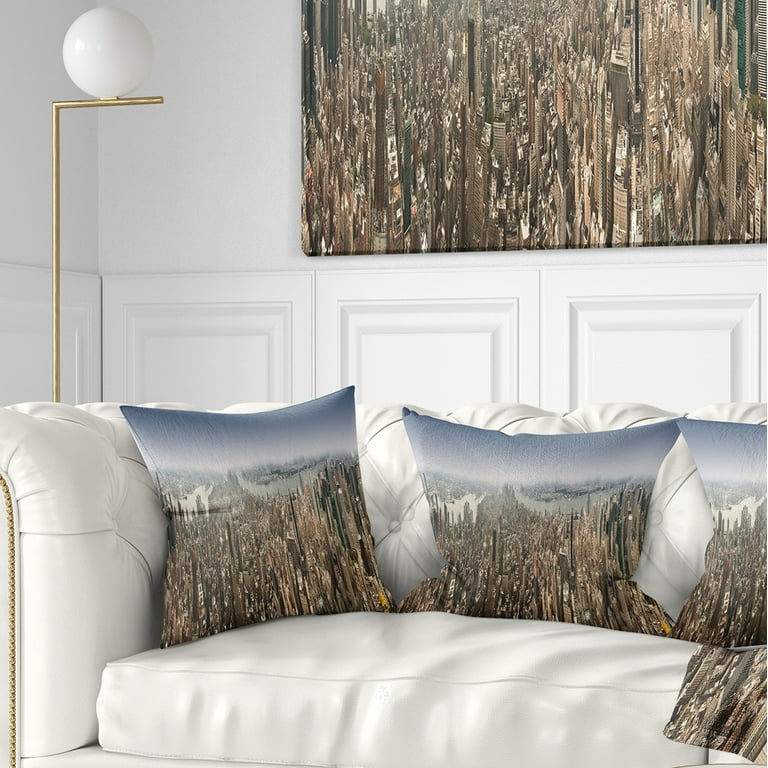This image depicts the modern living room of an apartment. The walls are predominantly white, accented with decorative wainscoting that features inlaid rectangular panels running halfway up the wall, creating a blend of contemporary and traditional aesthetics. On the left side of the room stands a sleek, modernistic lamp with a gold stand and a spherical globe atop it, suggesting it is a light fixture, though the room is brightly lit by daylight. 

A white, possibly leather, sofa occupies the bottom portion of the image, distinguished by quilted back and side panels, and golden rivets. The sofa holds three pillows, each adorned with a detailed image of a dense cityscape, reminiscent of a futuristic metropolis. Above the sofa hangs a large, unframed photograph displaying the same cityscape, creating a cohesive and visually striking theme. The room exudes a stylish fusion of modernity and nature-inspired elements, tying together urban imagery with classic paneling.